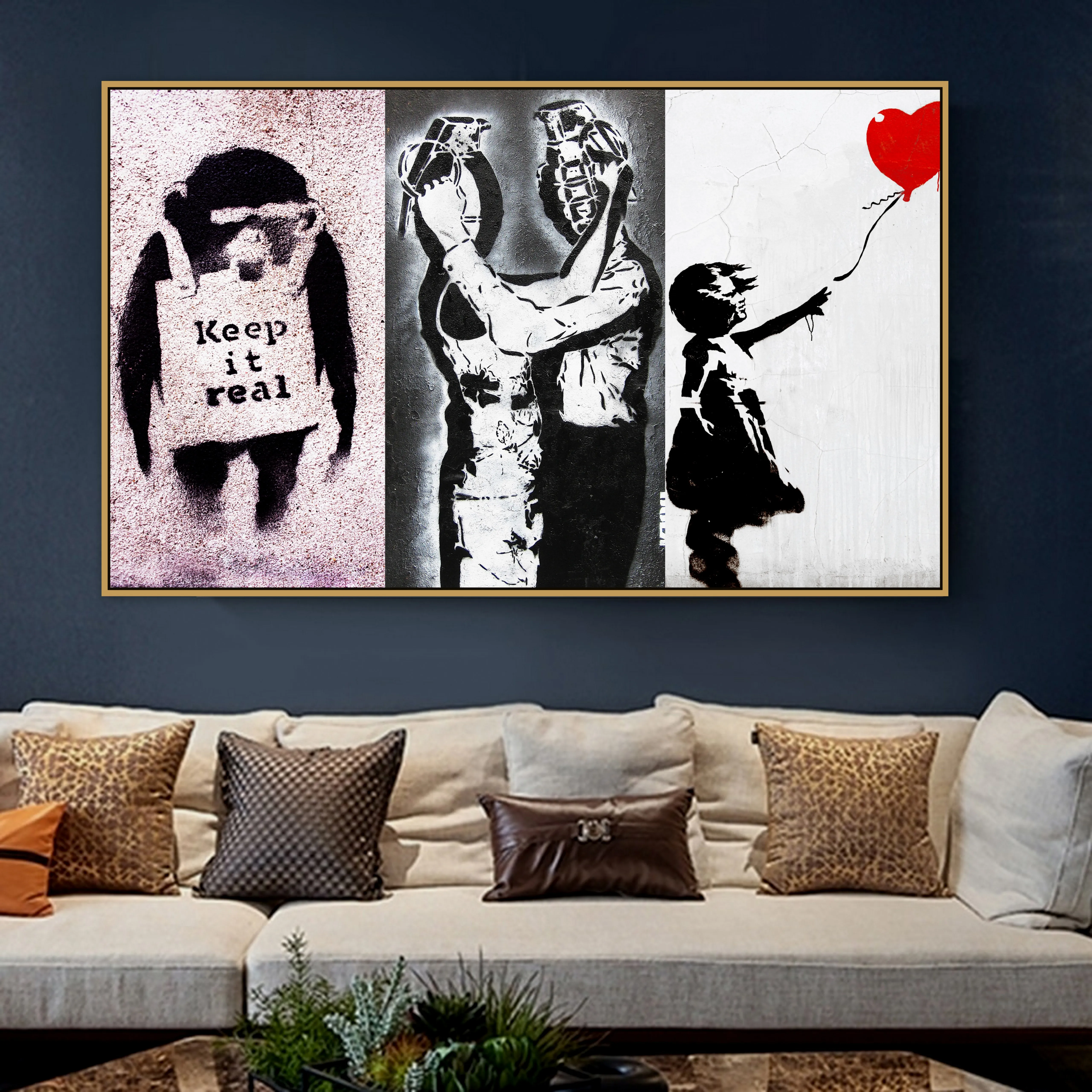The photograph captures a modern, neatly-arranged living room centered around a cream-colored sectional couch adorned with a variety of pillows in brown, golden, white, giraffe pattern, and checkered designs. In front of the couch, a sliver of what appears to be a shiny, potentially granite coffee table with green plants on top is visible. The backdrop is a rich, dark blue wall, almost denim navy in color. Dominating the wall above the couch is a large, framed artwork divided into three sections. The left segment features a whimsical illustration of a monkey wearing sunglasses with a sign that reads "Keep it real" around its waist. The middle segment depicts two humanoid figures embracing, their heads replaced by grenades, each poised to pull the other's pin. The right segment shows a child reaching for a red, heart-shaped balloon. The overall composition of the room combines modern aesthetics with intriguing artistic elements, creating a visually engaging and detailed setting.